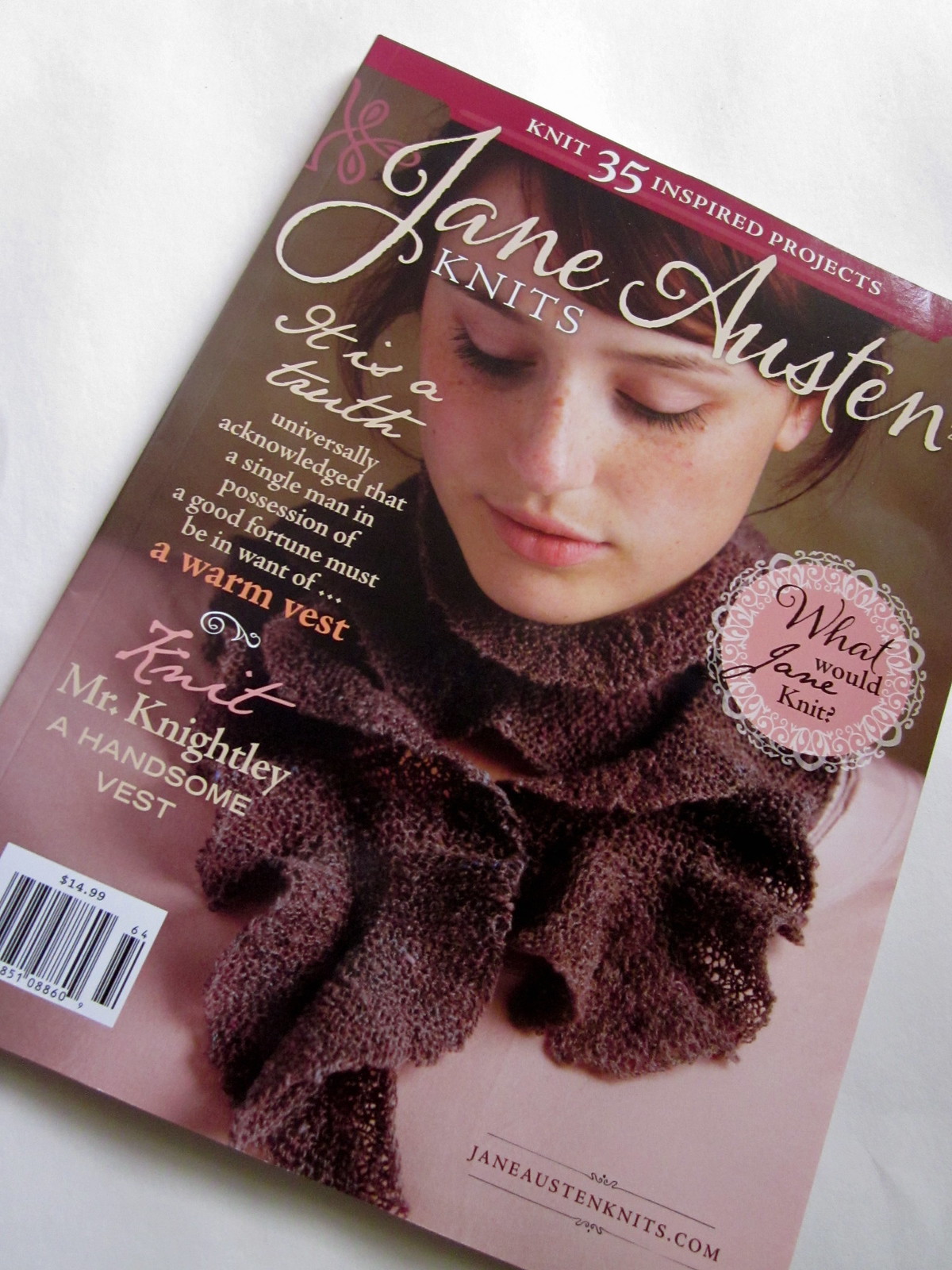The image features the cover of a magazine titled, "Jane Austen Knits," positioned on what appears to be a white cloth background, slightly tilted clockwise with the top right up and bottom left down. The top banner of the magazine is a maroon stripe reading "Knit 35 Inspired Projects." The title "Jane Austen" is elegantly written in yellow cursive, followed by "Knits" in smaller white font.

The cover showcases a young white woman with auburn hair, freckled skin, and partially obscured eyes as she looks down. She is wearing a vintage-style dark brown scarf over a pink garment. To her left, in various fonts, is the quote, "It is a truth universally acknowledged that a single man in possession of a good fortune must be in want of a warm vest. Knit Mr. Knightley a handsome vest."

Overlaying the image is a circular, doily-like design with the text "What would Jane knit?" in black. The bottom right corner features JaneAustenKnits.com in dark pink font, and a barcode is visible at the bottom left corner. The magazine is priced at $14.99.